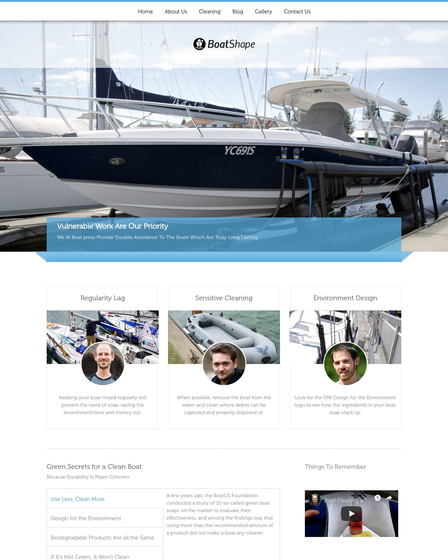This image showcases a web page dedicated to a boat cleaning business. The navigation menu is prominently displayed with links to "Home," "About Us," "Cleaning," "Blog," "Gallery," "Contact Us," and "Boat Ship," along with the business name. The page features images of boats, emphasizing the company's focus. A highlighted section reads, "Vulnerable work is our priority. We at Boat Press provide durable assistance to boats that is truly long-lasting." The site emphasizes their commitment to sustainable practices with phrases such as "Regularity log, sensitive cleaning, environment design, green secrets for clean boats because durability is a major concern," and "Things to remember: use less, clean more. Design for the environment. Biodegradable products are all the same. If it's not green, it won't clean."